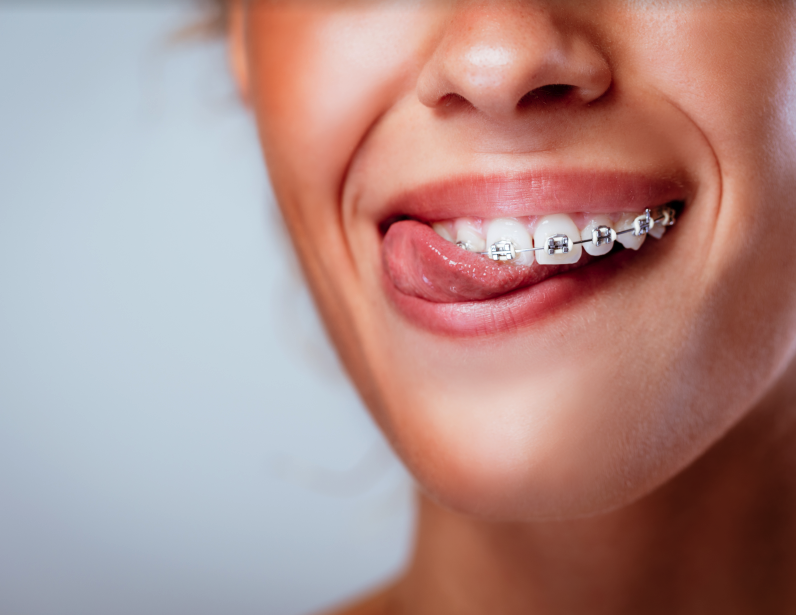This is a detailed close-up photograph, likely taken professionally, of a young woman smiling. The frame captures her face from just below the bridge of the nose down to the neck, with wispy brown hair partially visible. She has straight teeth adorned with white metallic braces. In the image, she is playfully rubbing the left side of her braces with her tongue, as though feeling them or making a funny face. The young woman is positioned towards the right side of the photograph, slightly smiling, and her Caucasian features are softly lit from either the top or head-on, enhancing the brightness of the imagery. The background is a plain, white wall, giving the photo a clean and minimalistic look. The focus on her mouth and braces could suggest that this image might be used as an advertisement for orthodontic services.